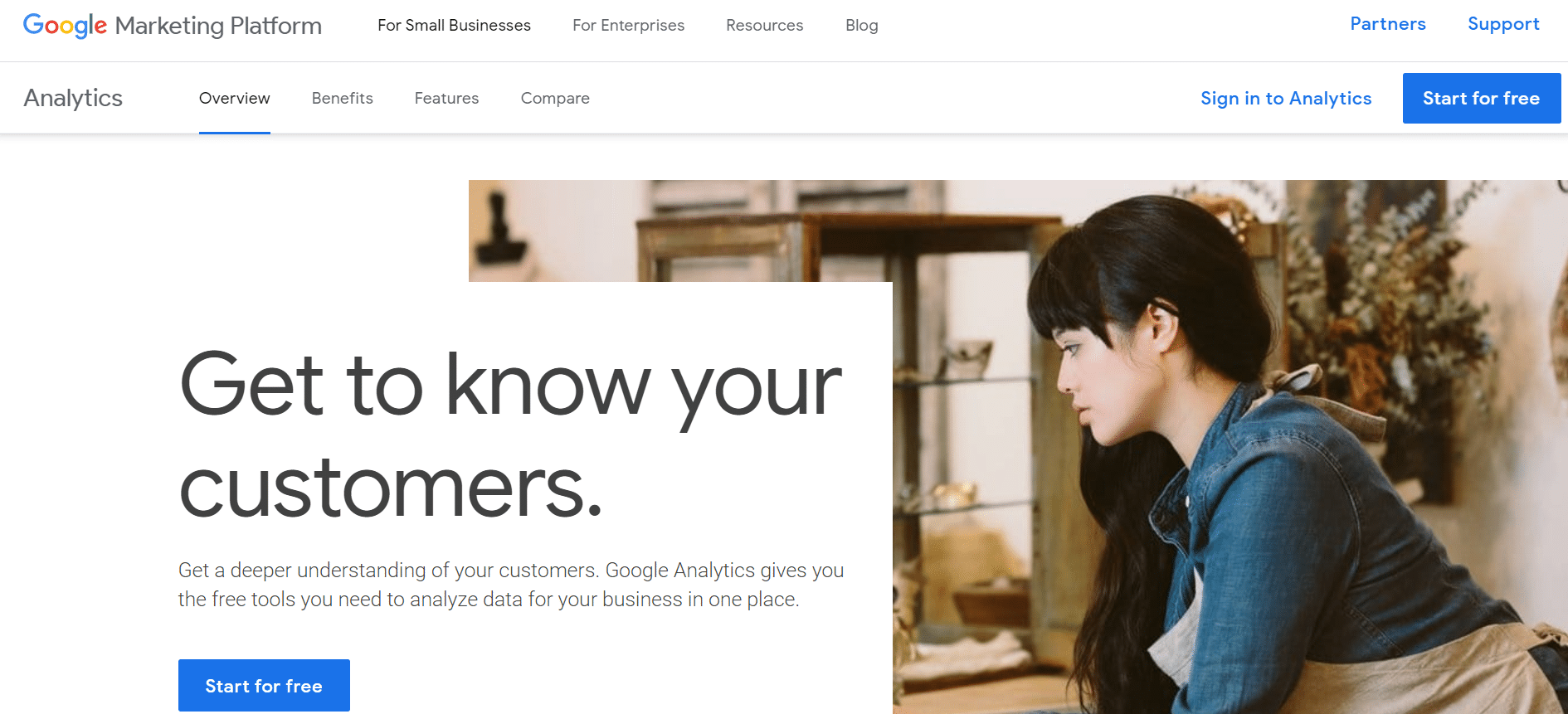A detailed, cleaned-up caption for the described image could be:

"The webpage for Google Marketing Platform prominently features the header text 'Google Marketing Platform' with subsections like 'For Small Business', 'For Enterprises', 'Resources', and 'Blog'. On the right side, navigation options include 'Partners', 'Support', 'Sign in to Analytics', and a blue 'Start for free' button. The main image shows a young woman, possibly wearing an apron, gazing downwards, suggesting she might be an artisan or craftsperson who owns a business. Accompanying text reads: 'Get to know your customers. Get a deeper understanding of your customers. Google Analytics gives you the free tools you need to analyze data for your business in one place.' The blue 'Start for free' button appears again below this text. This platform offers free tools for businesses to conduct marketing analytics, with an emphasis on understanding customer behavior. The image and the text together aim to represent small business owners who could benefit from using Google Analytics to improve their marketing strategies."